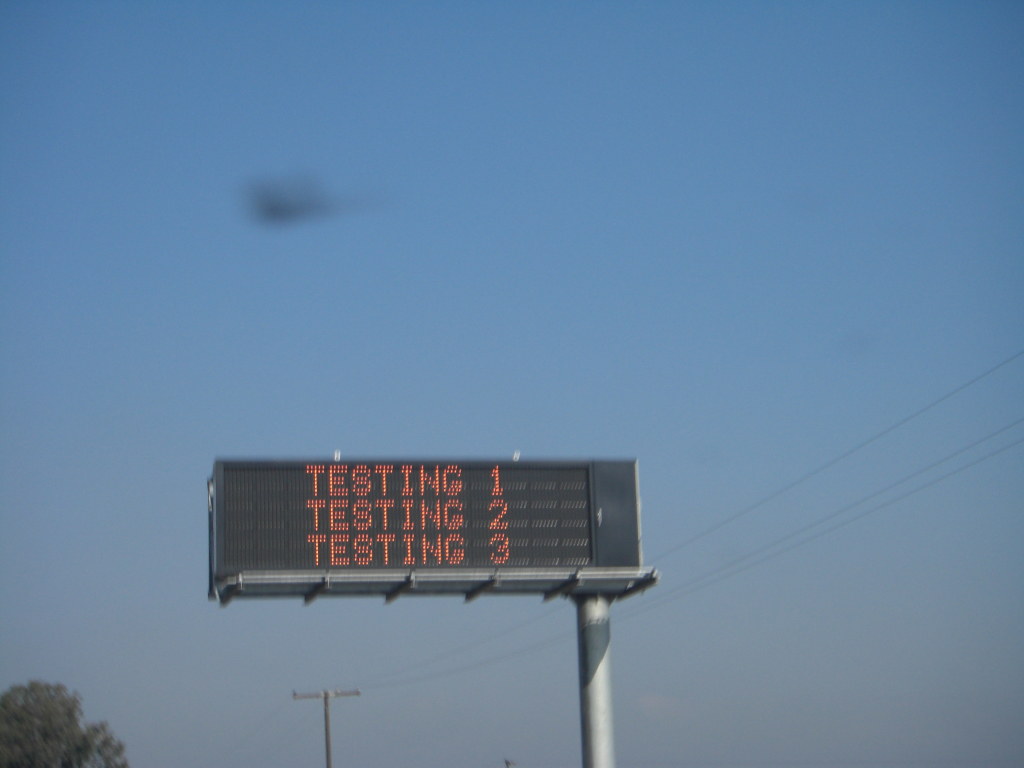The image showcases a vintage highway sign prominently displaying the text "Testing One, Testing Two, Testing Three" in bold red letters against a black background. The sign is mounted on a single pole situated on its right side. The surrounding scenery depicts a clear, deep blue sky, devoid of any clouds but with a slight haziness that adds an aged, nostalgic feel to the photograph. In the lower left corner, a solitary tree is partially visible, adding a touch of greenery to the scene. Additionally, a telephone pole and wires can be seen extending across the sky, contributing to the overall rustic aesthetic. There is also a nondescript blurry object in the distance, further enhancing the image’s vintage characteristic. The colors throughout the image appear faded and worn, accentuating the impression that this is an older photograph taken on a perfectly clear day.